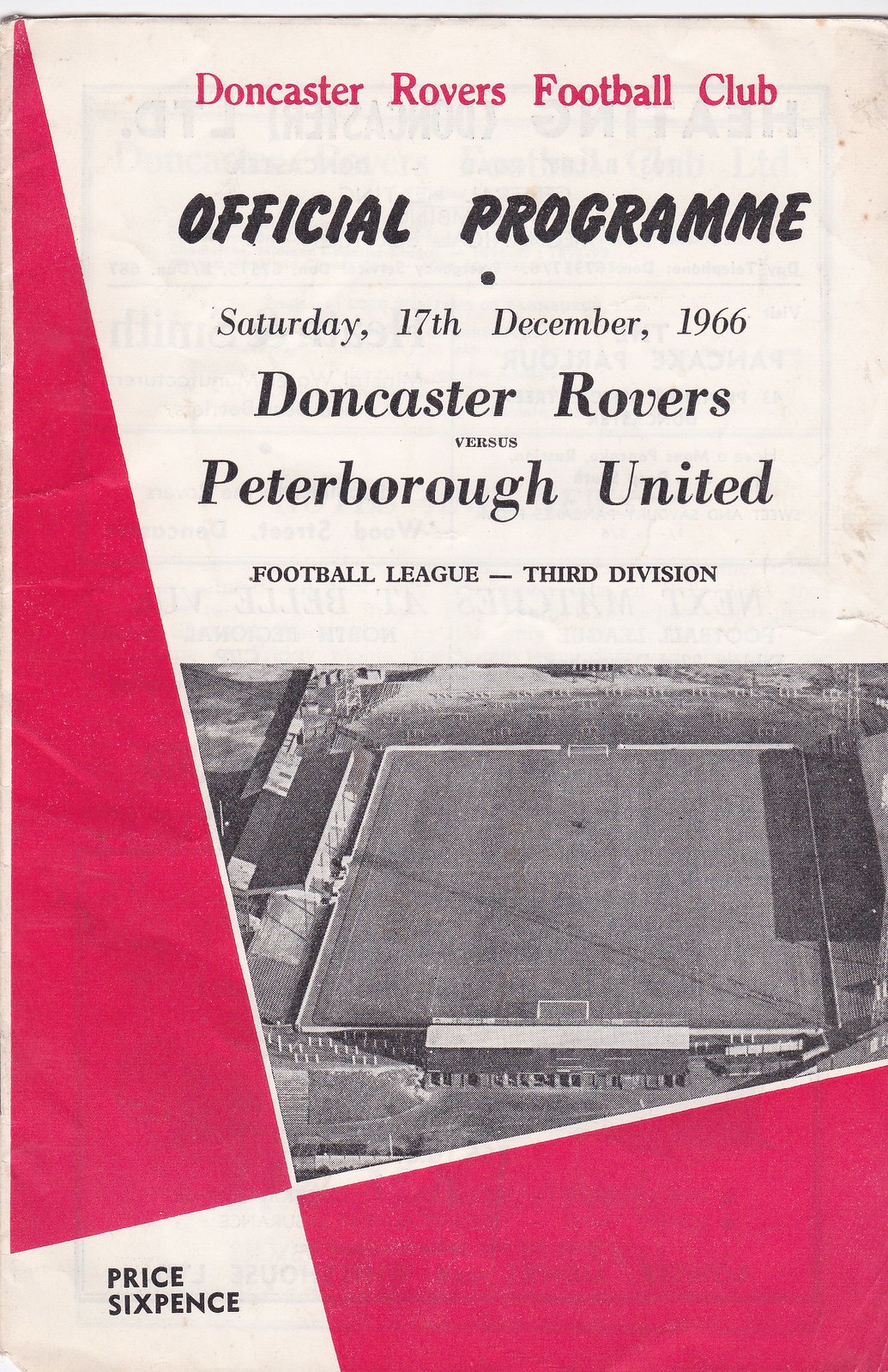This image is a vintage print publication cover from a football program, featuring a black-and-white portrait orientation with spot color in red. At the top, bold red letters announce "Doncaster Rovers Football Club." Below this, in bold black italic text, the words "Official Program" appear, followed by the lighter text "Saturday, 17th December 1966." The matchup "Doncaster Rovers vs. Peterborough United," identified as a "Football League Third Division" game, is printed in bold black text. A speckled black-and-white aerial photograph of a football field dominates the center of the cover, with a distinct red triangular pattern emerging from the top left and extending across the bottom right. In the bottom left corner, the price is marked in black text as "Price Sixpence." The scan reveals some barely visible internal text due to the lighting, but these words remain illegible.